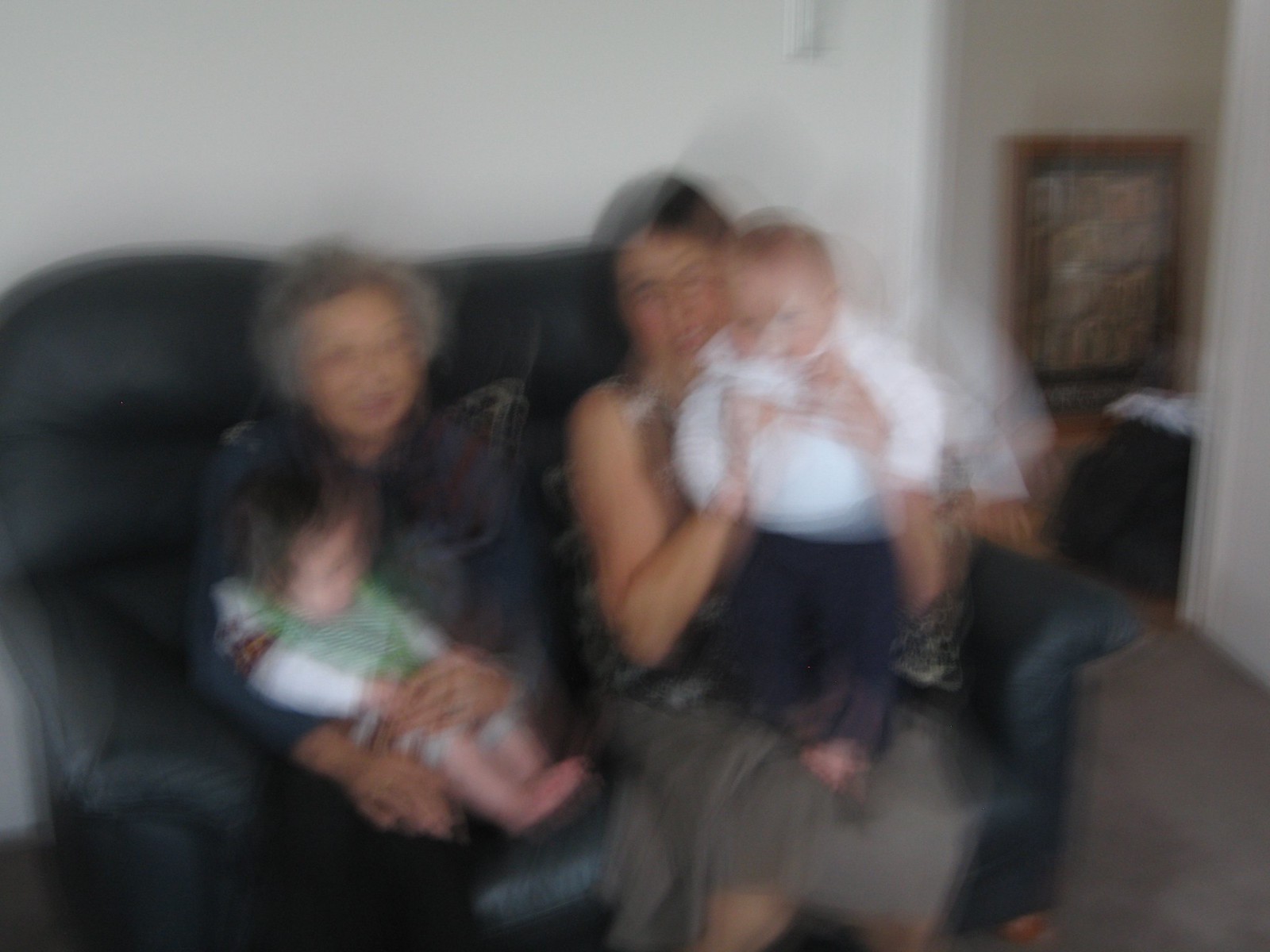The photograph is a color image in landscape orientation, capturing a slightly blurred scene inside a cozy living room. Dominating the foreground is a well-stuffed, blue loveseat with a glossy leather finish and wooden accents. Seated on the loveseat are two females and two young children. On the left, an elderly gray-haired lady tenderly holds a baby girl with dark hair, who is dressed in a green and white outfit. To the right, another female, clad in a strapless brown and white top paired with a gray skirt, cradles a little boy dressed in a long-sleeved white shirt and blue pants. Notably, both children are barefoot.

The background showcases a white wall and a gray carpet that extends across the living room floor. An open doorway leads to an adjacent room, which appears to be a bedroom. Part of the bed is visible through the doorway, alongside a piece of art adorning the wall, adding a touch of decor to the background scene.